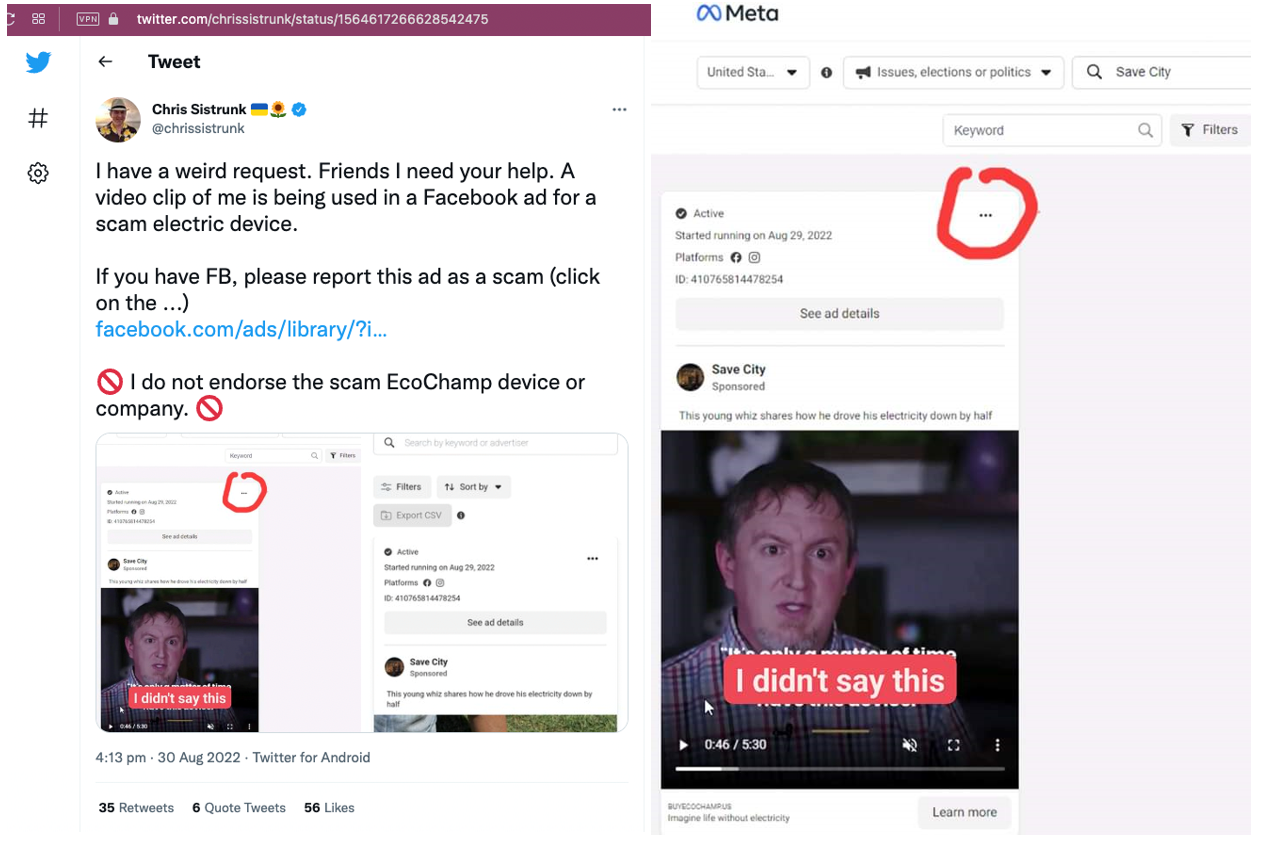The image features two juxtaposed screenshots. The left screenshot displays a Twitter interface. At the top-left corner, the familiar Twitter logo and icons for hashtags and settings are visible. Moving rightward, the "Tweet" button, followed by the profile of Chris Sistrunk, identifiable with an avatar alongside the Ukrainian flag and other icons, are displayed. The tweet reads, "I have a weird request, friends. I need your help. A video clip of me is being used in a Facebook ad for a scam electric device. If you have Facebook, please report this ad as a scam by clicking on the '...' (facebook.com/ad/library/question). I do not endorse the scam Eco-Champ device or company."

The right screenshot is a larger image, presumably from Facebook, focused on an ad. It indicates the ad is related to "Meta, Issues, Elections, or Politics," highlighting a segment with a dotted circle around the '...' menu icon. Details note that the ad became active on August 29, 2022, with a prompt to "See ad details" and a disclaimer: "I didn't say this."